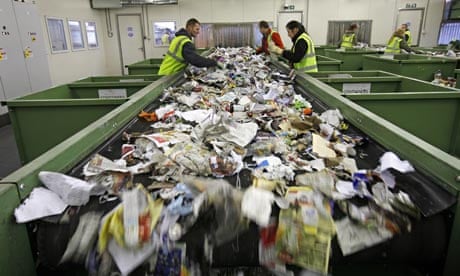This detailed image depicts the interior of a bustling recycling plant. Dominating the center is a long, black conveyor belt, laden with what appears to be recyclable paper and rubbish. The conveyor belt extends from the foreground to the back of the image, flanked by dark green dividers. Workers in high-visibility jackets of yellow or green, paired with variously colored sweatshirts, sort through the materials. To the left of the main conveyor belt, a worker in a yellow high-vis jacket is stationed, while on the right, another worker and a lady are engaged in sorting, both in high-vis jackets. Large green bins are placed next to them for collected materials.

In the background, a similar setup is visible with another conveyor belt and three additional workers in high-visibility jackets. To the right side, the scene is framed by white walls with three window panels. On the left, the space includes gray lockers against a light-gray wall, enhancing the industrial feel of the environment. Overall, the image captures the essence of a busy work environment dedicated to recycling, with workers methodically processing the incoming waste materials.